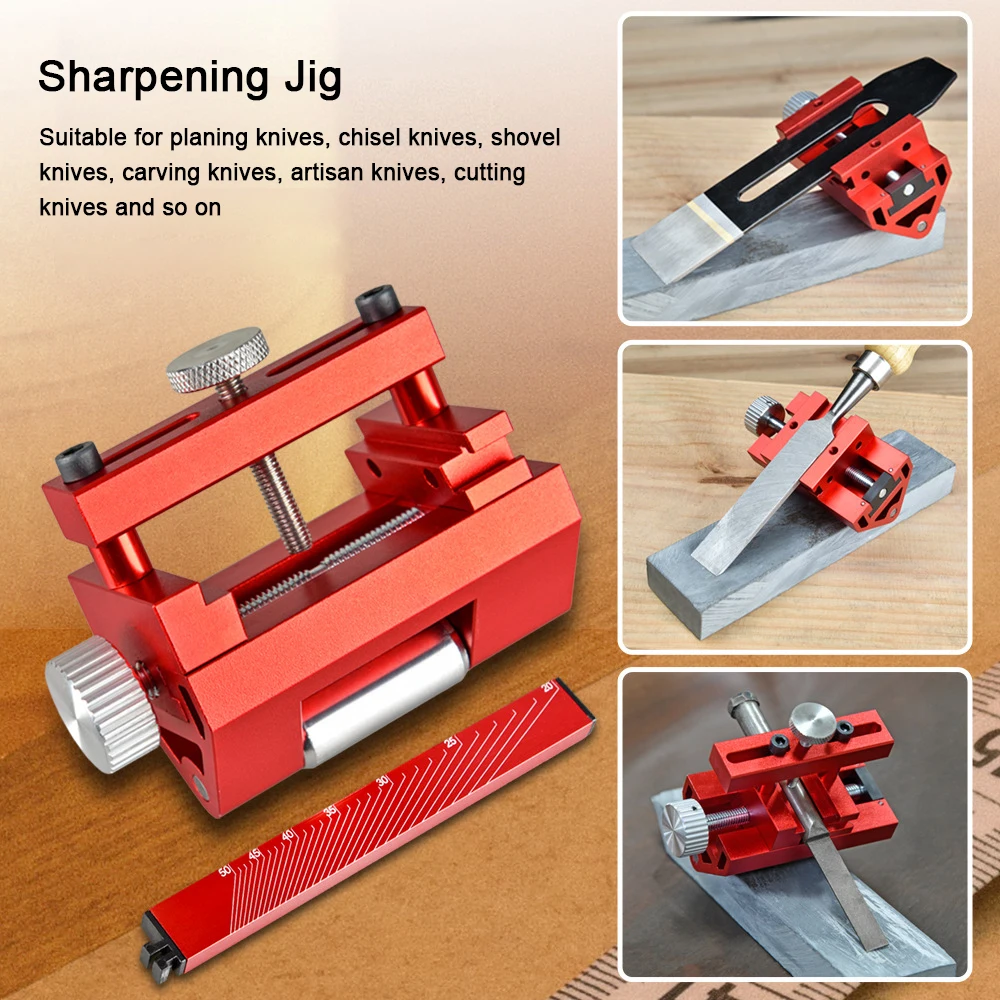The image showcases a metal sharpening jig prominently featuring red and silver components, including adjustable knobs. The large central photograph of the jig occupies most of the image's left side, displaying the jig set against a wooden surface with a wooden ruler in front of it. In the image's background, there is a text overlay stating, “sharpening jig, suitable for planing knives, chisel knives, shovel knives, carving knives, artisan knives, cutting knives, and so on.” On the right side of the image, there are three smaller stacked photos showing the sharpening jig in action. The top thumbnail displays the jig sharpening a black item, the middle one features it sharpening a chisel, and the bottom thumbnail shows it honing what appears to be an artisan knife, with all these tools being worked on a whetstone placed on a wooden surface.